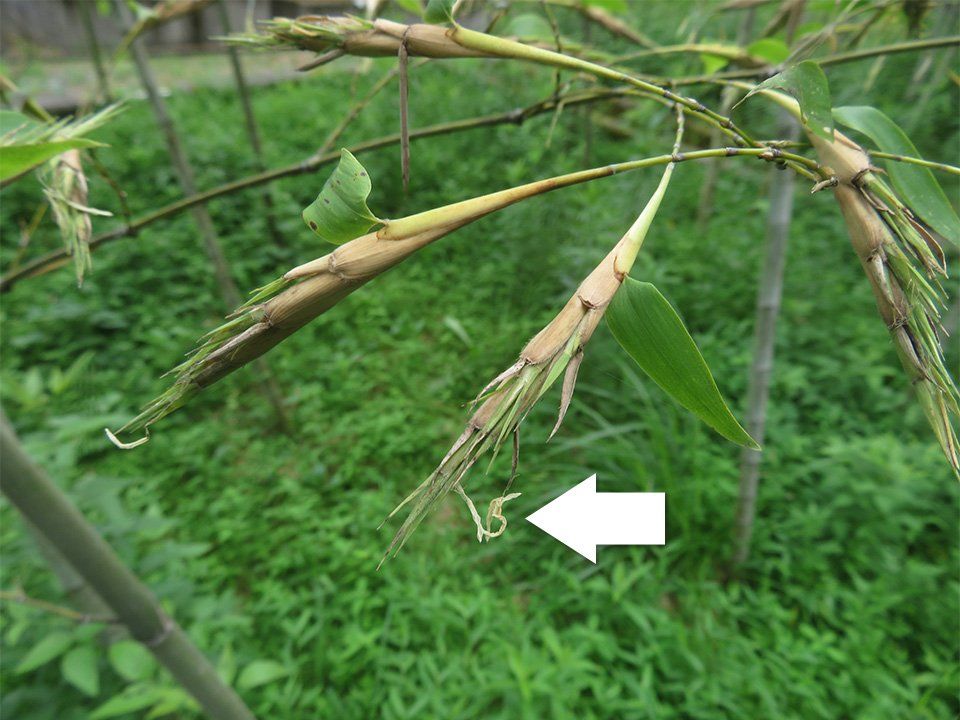The image, taken outdoors during the day, prominently features bamboo trees planted with ample space between each. These trees rise from a landscape of shorter, vibrant green vegetation. The central focus of the photograph is the growing shoots or branches of the bamboo, particularly the tips adorned with fresh green leaves and buds. A white arrow highlights a particular tip of one of these branches, pointing to a small, whitish, stringy entity that resembles a coiled worm. Whether this entity is part of the plant or a parasite is unclear. In the background, you can discern additional branches, green leaves scattered close to the soil, and a house with gray walls and black trim, partially obscured by the lush greenery. The house is fronted by a concrete sidewalk and framed by a silver metal garden gate. The overall scene is serene and natural, with vivid green hues and no significant disturbances.